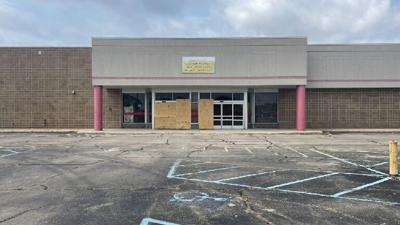This photograph captures a dilapidated outdoor scene featuring what appears to be a closed or abandoned building, possibly a supermarket or shopping mall. The structure has a flat-topped facade held up by two prominent pink pillars and displays a largely indiscernible sign with a white top and yellowish-green bottom. The building's exterior is a mix of brown and gray tones, with the left side showcasing a brown, plaid-like pattern. Many of the windows are broken and covered with plywood, particularly the front doors on the left.

In front of the building, the neglected parking lot is visible, marked by tire imprints and extensive dirt and debris. Chalk writings are scattered on the ground. A yellow stopping post and a designated handicapped parking space can be seen to the right side of the image. The sky above is clear with white clouds, giving a sense of contrast to the deteriorating scene below.